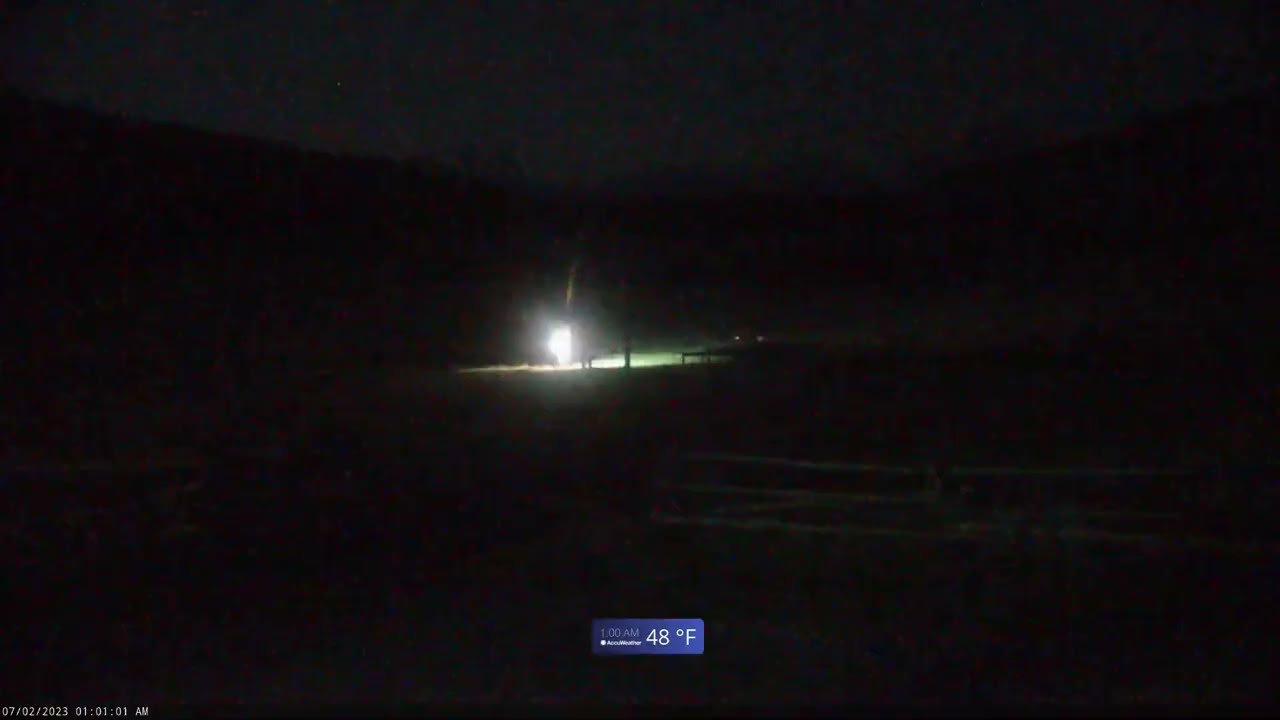This nighttime scene, shrouded mostly in darkness, appears to be a screen capture from a video, possibly a news segment. The only significant light source in the image is a vivid light in the center, which could be from fireworks or an explosion, illuminating the surrounding grass and casting faint shadows. Despite the general obscurity, a metal fence and faint human figures can be discerned in the dim light. The horizon reveals vague shapes of hills and a division between the night sky and the terrain. At the bottom of the image, a caption within a blue rectangle indicates it is 1 a.m. with a temperature of 48 degrees Fahrenheit. Additional text includes a timestamp, "07-02-2023, 01:01:01 AM".